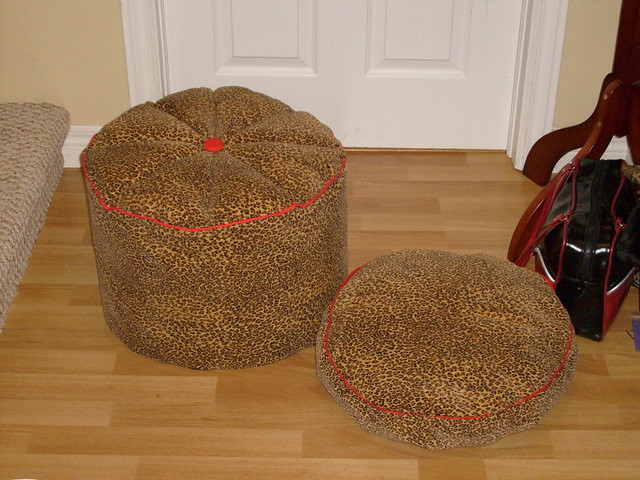The photograph captures an interior space, likely a porch area of a house, featuring two prominent pieces of leopard print furniture on a wooden plank floor with varying shades of wood grain. At the center, there is a circular leopard print ottoman or puffet, detailed with a red trim around the top and a red button in the middle, suggesting a cushioned seat. Beside it lies a matching detachable cushion, indicating it might have come off the top of the ottoman. The distinct red trim and button on both pieces enhance their visual coherence. To the left, a gray couch is partially visible. The room also includes a white door with white molding and a tan-colored wall. At the upper right, a wooden coat rack stands next to a small dark brown leather satchel with light brown handles. Additionally, the lower left corner reveals the first step of a carpeted staircase. Finally, a black, maroon, and white overfilled case or potentially a gym bag is placed near the bottom center, adding to the scene's lived-in feel.